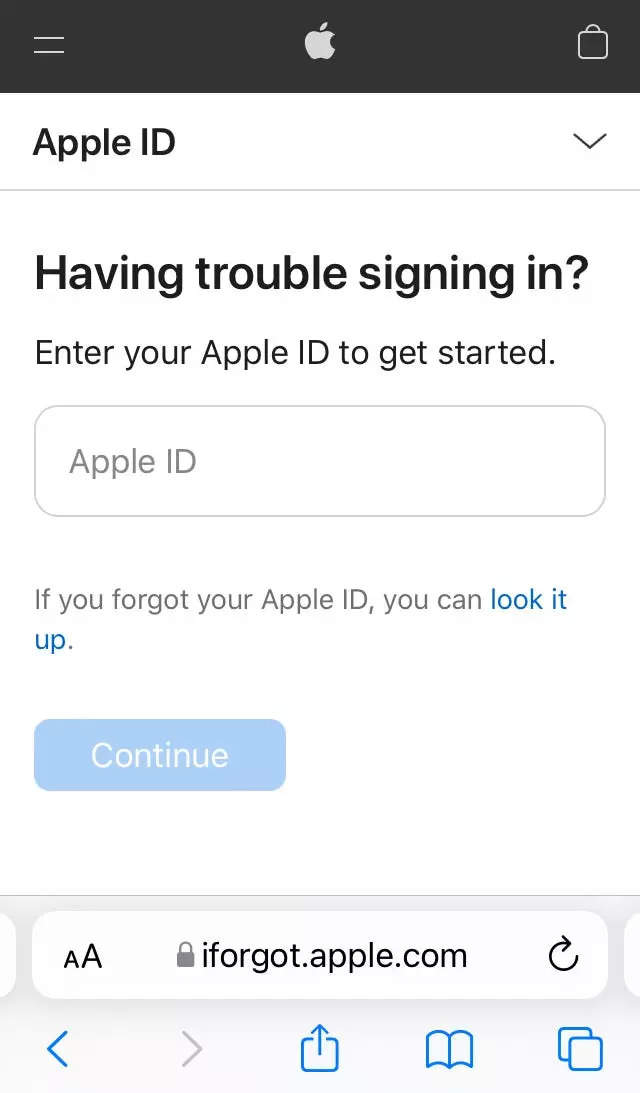The image is an Apple interface illustration focused on the Apple ID sign-in process. At the top, a black bar frames the scene. Central to the image is the iconic white Apple logo, flanked by a box on the right and two lines on the left, symbolizing Apple’s design elements. Below this, the bold, black text "Apple ID" is prominently displayed with a downward arrow indicating further information below.

The main section of the image features a large text bar, where instructions in bold black text read, "Having trouble signing in?" This is followed by the prompt, "Enter your Apple ID to get started," accompanied by a white text field labeled "Apple ID" for user input. Additionally, there's a clickable blue text link, "look it up," for users who have forgotten their Apple ID, leading them to further assistance.

Beneath the input field, a blue "Continue" button invites the user to proceed. The lower part of the image presents an example search bar showcasing the URL "iforgot.apple.com," with a lock icon for security, two text size adjustment A’s on the left, and a circular arrow on the right for refreshing the page.

At the very bottom, navigation arrows are displayed: a blue arrow pointing left and a gray arrow pointing right, indicating backward and forward navigation options. Supplementary icons, including a download symbol, a book symbol, and two overlapping squares, further enrich the image's functional and illustrative context.